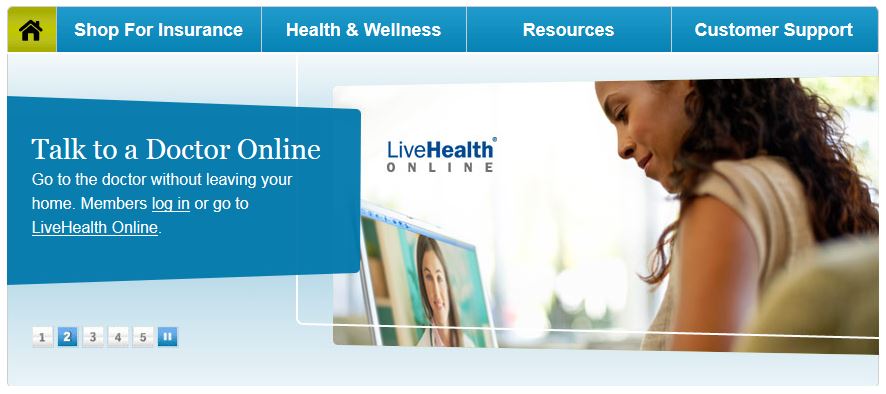The image appears to be a screenshot of a webpage, displayed in a rectangular format. At the top of the page, there is a blue border. Below this border, a navigation menu is divided into five sections, separated by thin white lines. The first section on the left is a yellowish-green block featuring a house icon, indicating the "Home" section. The next four sections, with their first letters capitalized, are labeled "Shop for Insurance," "Health & Wellness" (with an ampersand symbol), "Resources," and "Customer Support."

In the main content area, there is a prominently displayed message reading "Live Health Online," with the word "Health" emphasized in bold text. Below this message, there is an image of a woman with long, curly dark hair, looking at a screen that shows an image of a female doctor.

To the right of this image is a darker blue rectangular block superimposed on the "Live Health Online" message. This block contains white text that reads: "Talk to a doctor online. Go to the doctor without leaving your home." Below this message are the underlined options "Members log in" and "Go to Live Health Online."

At the bottom left of the page, there is a row of page numbers for navigation.